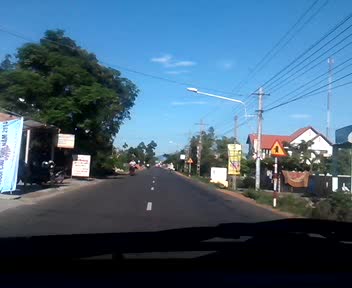Captured through the pristine front windshield of a truck cab, this photo reveals a serene two-way road with clear, white-dashed lane dividers. On the left side of the road, a pedestrian is seen walking midway down the lane, flanked by a variety of storefronts and street signs, some adorned with banners. Towering trees and lush greenery enhance the left side’s vibrant atmosphere, while the expansive blue sky provides a serene backdrop.

To the right, white poles supporting black power cables line the street alongside several white streetlights. Red and white poles display triangular-shaped signs with a yellow inset, depicting a figure extending a hand. In the distance, a large white house with a terracotta roof peeks through the greenery, surrounded by verdant tropical plants. Additional signs along the power lines suggest a well-signposted area, characteristic of a tropical region. The bottom of the frame captures the truck’s dashboard and windshield wipers, completing this detailed roadside panorama.